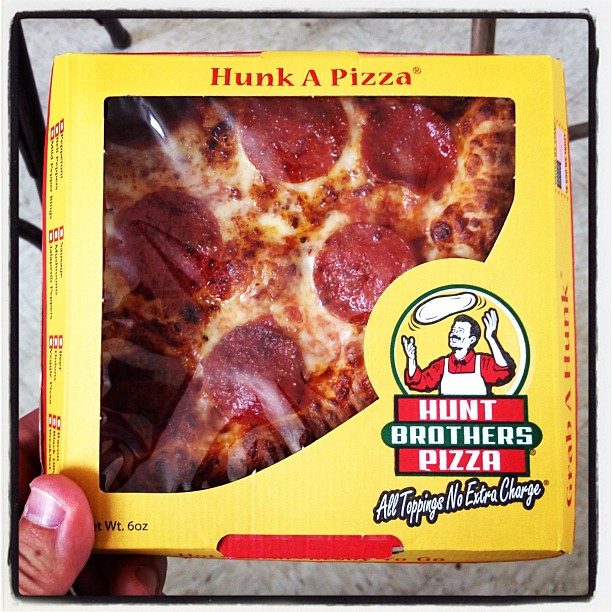This image depicts a yellow square pizza box with a clear window through which a cooked pepperoni pizza is visible. A person's thumb is seen holding the box in the bottom left corner. The box features the text "Hunk a Pizza" in red along the top edge. On the bottom right, a logo illustrates a man wearing a red shirt, black bow tie, and white apron, with black hair and a mustache, tossing a circle of pizza dough above his head. The logo has a background of red and green stripes, with "Hunt Brothers Pizza" written in white against the green stripe. Beneath that, it reads "All toppings, no extra charge" in white text. Next to the thumb, the box indicates a net weight of 6 ounces.